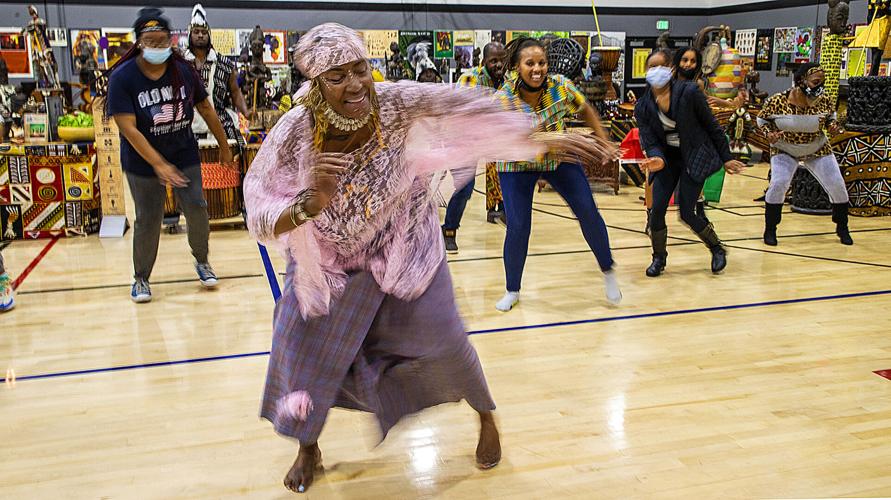This vibrant photograph captures an African dance class in mid-movement, led by an older black woman radiating joy. The woman, positioned at the forefront, is eloquently dressed in a light pink lacy shirt and a plaid skirt, accented by traditional African makeup and jewelry, including colorful necklaces and beaded wristbands. She dances barefoot on a light-colored hardwood floor, her outstretched arm slightly blurred, emphasizing her graceful motion. Behind her, a diverse group of dancers, primarily women of African descent, join in, some adorned in traditional African attire and others in casual American clothing, such as jeans and an Old Navy shirt. All participants appear relaxed and joyful as they follow the leader's movements. The backdrop features an array of African masks, symbols, textures, and colors, suggesting a culturally rich setting. Additionally, a man dressed in African garments plays a traditional drum, enhancing the authenticity of the dance experience. The overall energy of the scene is lively and celebratory, encapsulating the spirit of communal dance.